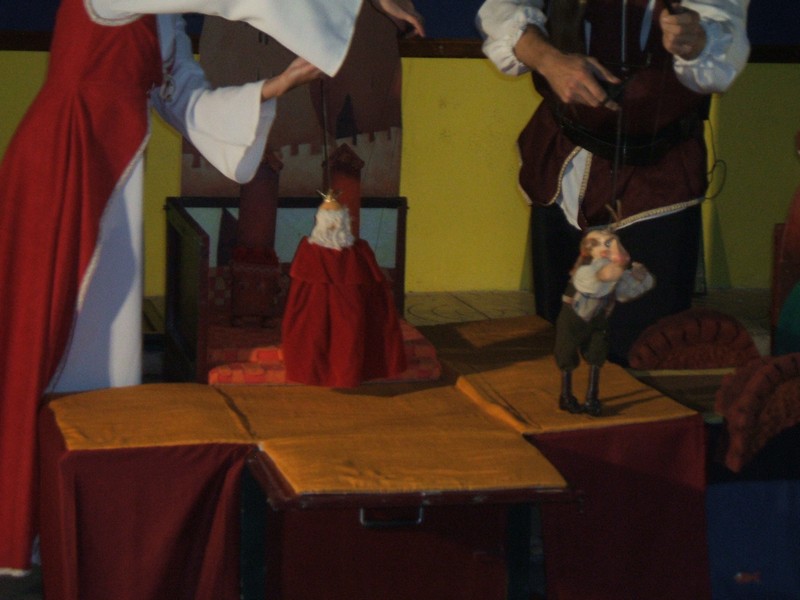The photograph captures a colorful and intricate scene of a stage performance featuring two string-controlled puppets. The image is slightly blurry, focusing on two puppeteers, whose faces are not visible, suggesting they are of European descent. On the left, a woman dressed in a deep maroon robe with flare white sleeves, is controlling a puppet of a king adorned with a white beard and royal attire. The man on the right, wearing a white shirt with ruffled sleeves, a dark brown vest, and black pants, is maneuvering a puppet attired in knickers, long stockings, and black shoes. Behind them, a yellow-walled background with a cardboard castle can be seen, enhancing the storytelling atmosphere. The puppets are positioned on a stage, which is covered with a cloth that appears to be dark purple or burgundy and brown, reinforcing the portable and foldable nature of the setup. The scene is vibrant and steeped in traditional puppet theatre aesthetics.